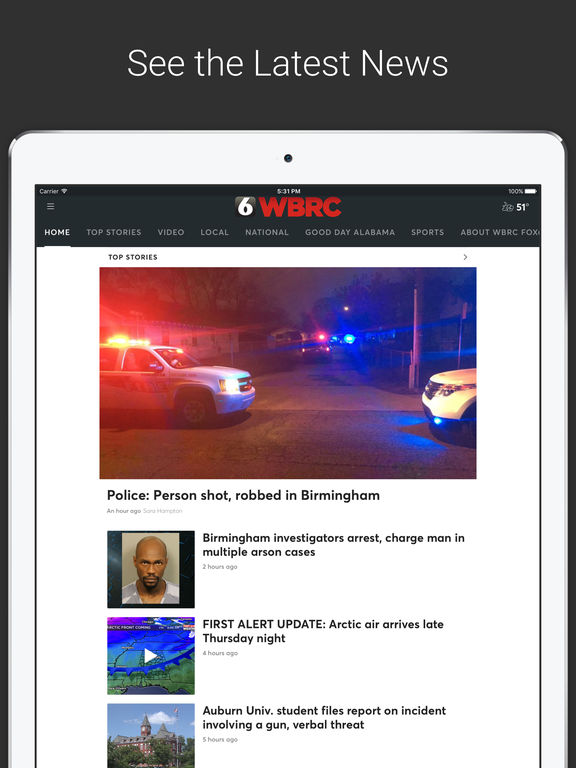This screenshot captures a news website, identified as WBRC, evidenced by the site’s name and logo displayed prominently at the top center of the page. The logo has a red background with a black section to the left that houses a white numeral "6," indicating the affiliation to WBRC 6 News. 

The image, though small, seems to be a promotional graphic for the website or its mobile app. The layout suggests a view outside a phone's screen. At the very top of the screenshot, a bold statement reads "See the latest news," creating a call to action. Positioned below this is a cutout illustration of a white smartphone displaying various informative texts and imagery, reinforcing the idea that this could be an app interface or a mobile website view. 

The phone’s screen shows details like the time, which appears as 6:31 or 5:31 p.m., along with a battery status symbol at 100% and a weather update indicating a temperature of 51 degrees, providing contextual information about the locale. 

Prominently featured are the top news stories, headlined by "Police: Person shot, robbed in Birmingham." Subsequent headlines include "Birmingham investigators arrest, charge man in multiple arson cases," "First Alert Update: Arctic Air arrives late Thursday night," and "Auburn University student files report on incident involving a gun, verbal threat." These headlines illustrate a mix of crime, weather updates, and campus safety reports, reflecting the variety of content available on the WBRC news site.